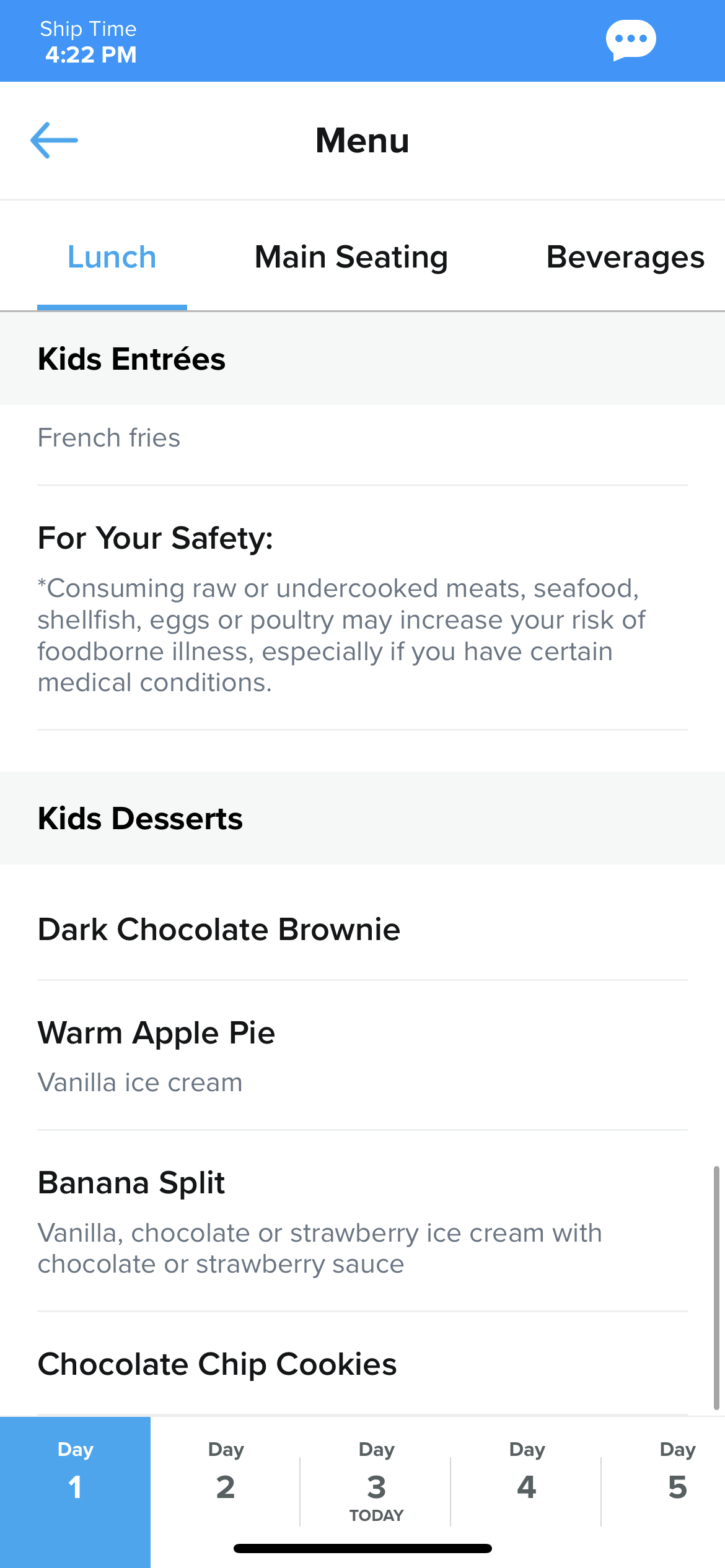In this image, we see a screenshot featuring a light blue banner spanning across the top. The banner displays white text on the left side that reads "Shift Time: 4:22 PM." Beneath this text, a blue arrow points to the left. To the right of the arrow, in black text, it reads "Menu." 

Below the banner, the menu items are listed from left to right. The first category, "Lunch," is highlighted in blue text, followed by "Main Seating," and "Beverages" in black text. Under the "Lunch" section, various items are listed, starting with kids' entrees and side dishes, such as French fries. 

A safety disclaimer in black text alerts diners: "For your safety, consuming raw or undercooked meats, seafood, shellfish, eggs, or poultry may increase your risk of foodborne illnesses."

Moving further down, items under "Kids Desserts" are detailed, including:
- Dark Chocolate Brownie
- Warm Apple Pie
- Vanilla Ice Cream
- Banana Split (with options of vanilla, chocolate, or strawberry ice cream, topped with chocolate or strawberry sauce)
- Chocolate Chip Cookies

The screenshot concludes with a blue square box containing the text "Day One."